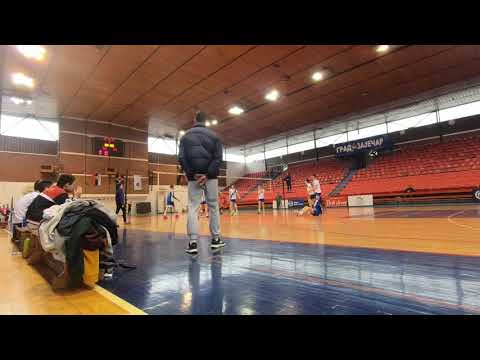This photograph captures a volleyball game taking place inside a large gymnasium with brown walls and red stands along the right side wall. The wide-angle shot, taken from a considerable distance, shows a volleyball net set up in the middle of the gym, with a group of about four players visible on one side. The scene includes a bench on the side stacked with uniforms or clothes, occupied by individuals who do not appear to be players. In the foreground, a man wearing blue jeans and a winter jacket stands watching the game, blocking most of the scene. Above the stands, large windows let in light, and a blue sign is visible, though the text is unreadable. A scoreboard hangs in the upper reaches of the gym, yet no information can be discerned from it. The sparse attendance in the stands suggests this might be a practice session rather than an official match.